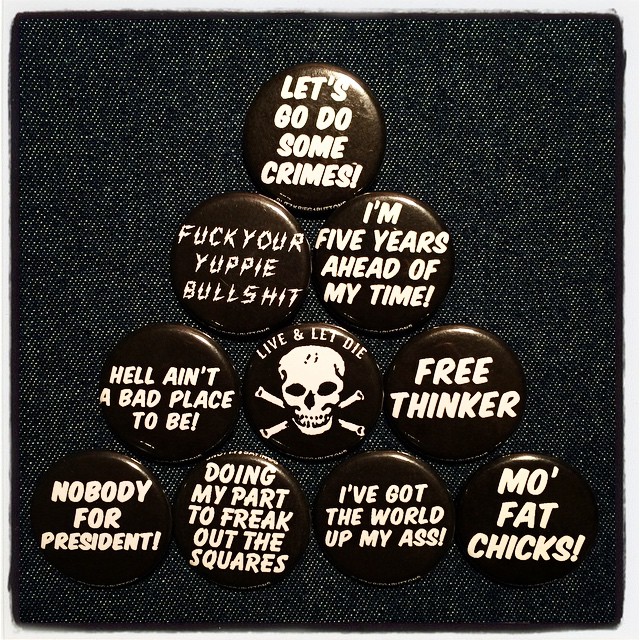The photograph captures a collection of black pin-on buttons adorned with white text, meticulously arranged in a pyramid shape atop a dark indigo or black denim background. The buttons, imbued with a punk aesthetic, convey an array of rebellious and provocative slogans. Starting at the apex of the triangle, the button reads "Let's go do some crimes!" Moving down to the next row from left to right, the buttons declare "Fuck your yuppie bullshit" and "I'm five years ahead of my time." The following row, consisting of three buttons from left to right, proclaims "Hell ain't a bad place to be," "Live and die in a skull shape" (accompanied by a skull and crossbones), and "Free thinker." The bottom row, also from left to right, features buttons that state "Nobody for president," "Doing my part to freak out the squares," "I've got the world up my ass," and "Mo' fat shit chicks." All the buttons share a consistent design of white lettering on a black background, emphasizing their uniformity and bold messages.